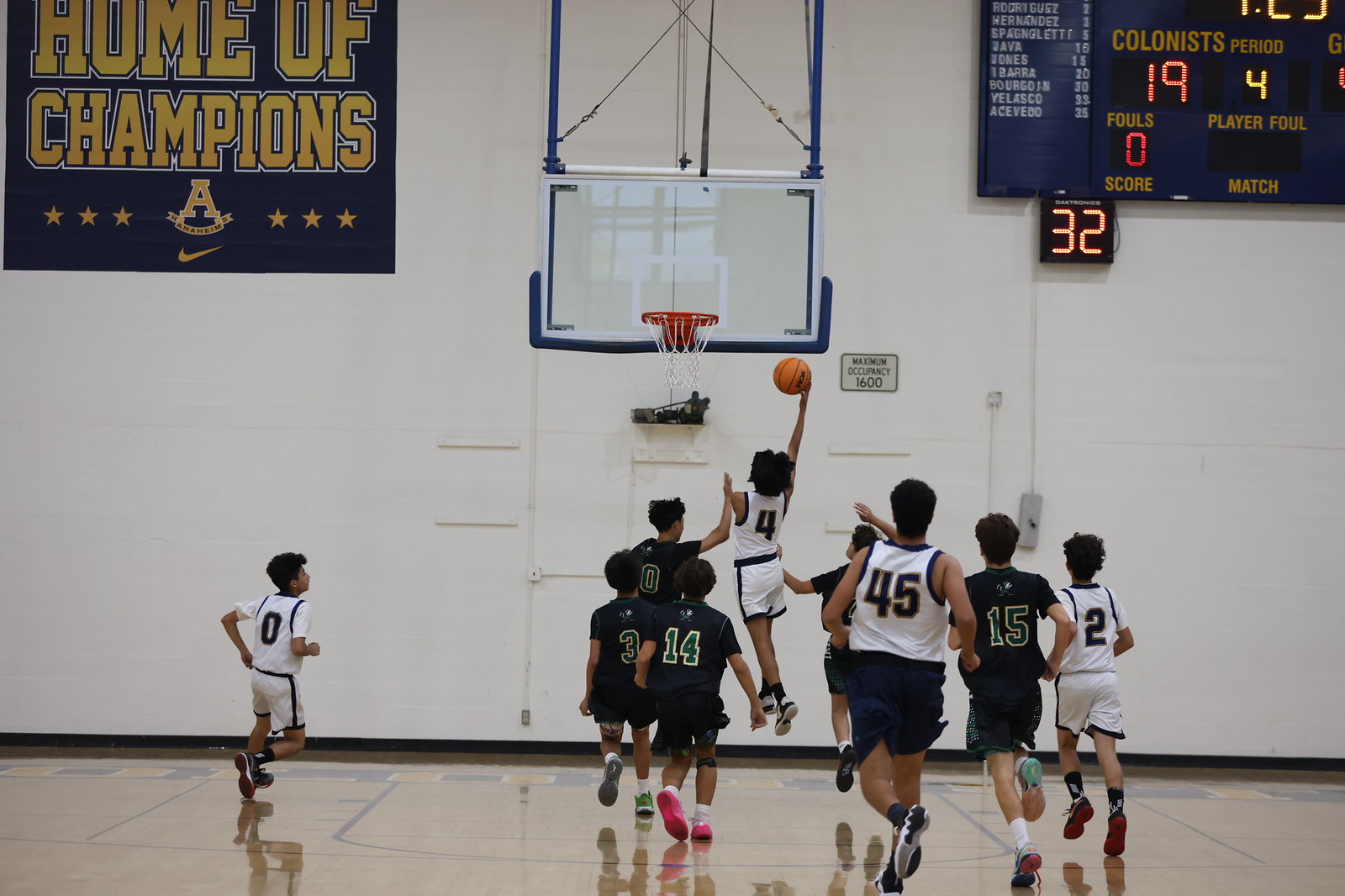In a brightly lit gymnasium with polished wood floors, middle school boys are engaged in an intense basketball game. The gym's white concrete block walls are adorned with a banner in the upper left reading "Home of Champions" and a maximum occupancy sign for 1,600 people. One team is dressed in white jerseys, while the other wears predominantly black uniforms. Player number four on the white team is airborne, poised to slam dunk the basketball towards the hoop suspended from the ceiling with a glass backboard. Surrounding him, players are sprinting in the heat of the moment. Several player numbers are visible, including zero, three, 14, four, 45, 15, and two. The high-mounted scoreboard on the upper right corner displays the home team's name, "Colonists," with 19 points, in the fourth period with no fouls recorded. Despite the visible excitement on the court, the stands are not shown, leaving it unclear whether this is a game with an audience or a practice session.